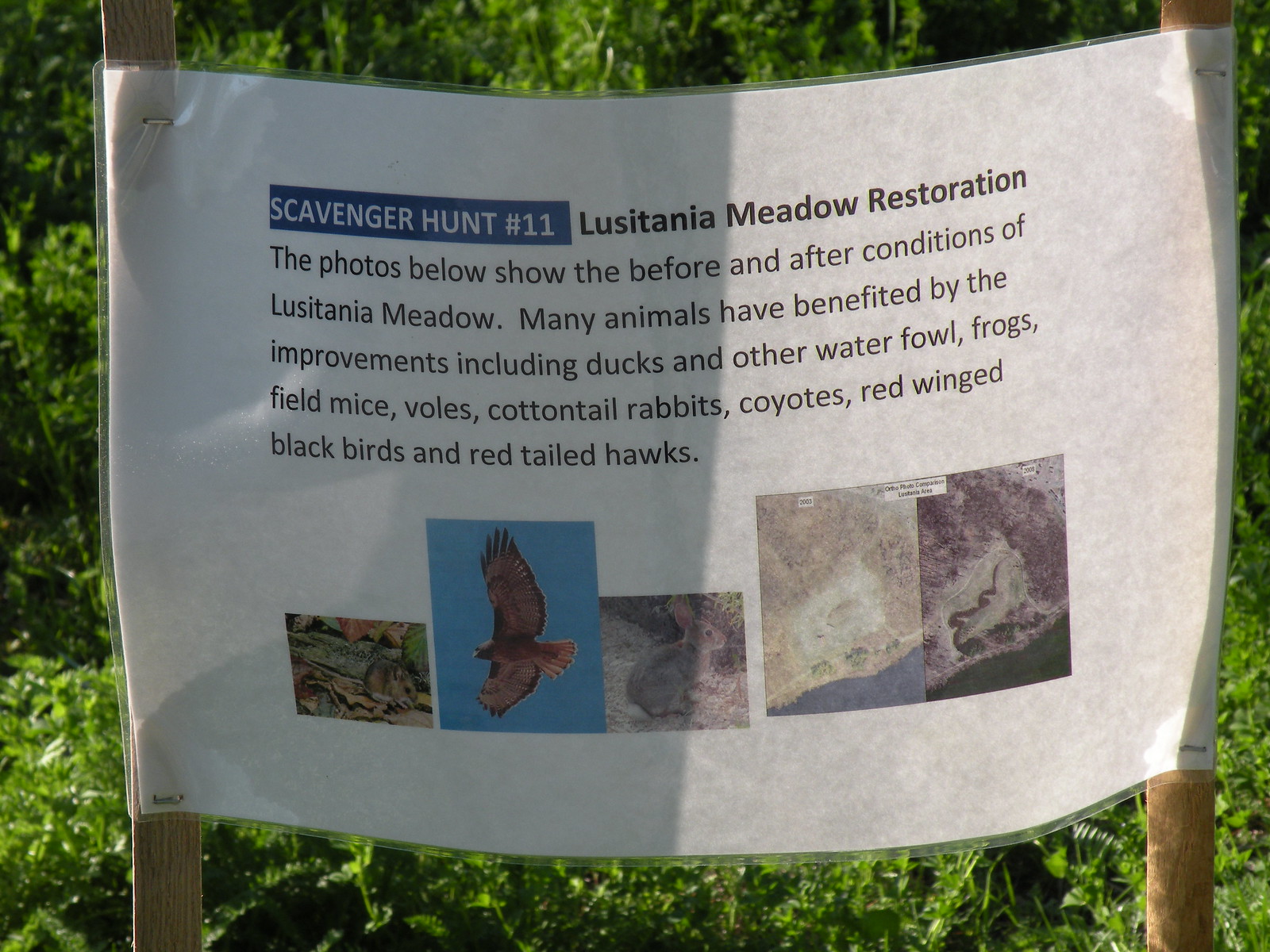In this vibrant color photograph taken outdoors on a sunny day, a laminated white sign is prominently displayed, stapled to two wooden poles amidst lush, green shrubbery. The sign, horizontally oriented, features a blue rectangle in the upper left corner with white text that reads "Scavenger Hunt Number 11". To the right, bold lettering announces "Lusitania Meadow Restoration". Below this title, the text explains that the photos beneath show the before and after conditions of Lusitania Meadow, highlighting the significant environmental improvements. The meadow's rejuvenation has notably benefited various animals, including ducks, other waterfowl, frogs, field mice, voles, cottontail rabbits, coyotes, red-winged blackbirds, and red-tailed hawks.

Encompassing five small, detailed photographs, the sign visually depicts these changes. One image appears to show a little mouse, another a large bird, and a third features a rabbit. There's also what seems to be an aerial view of the meadow, showcasing its transformation highlighted by an expanse of very green grass and possibly weeds, illustrating the thriving natural habitat.